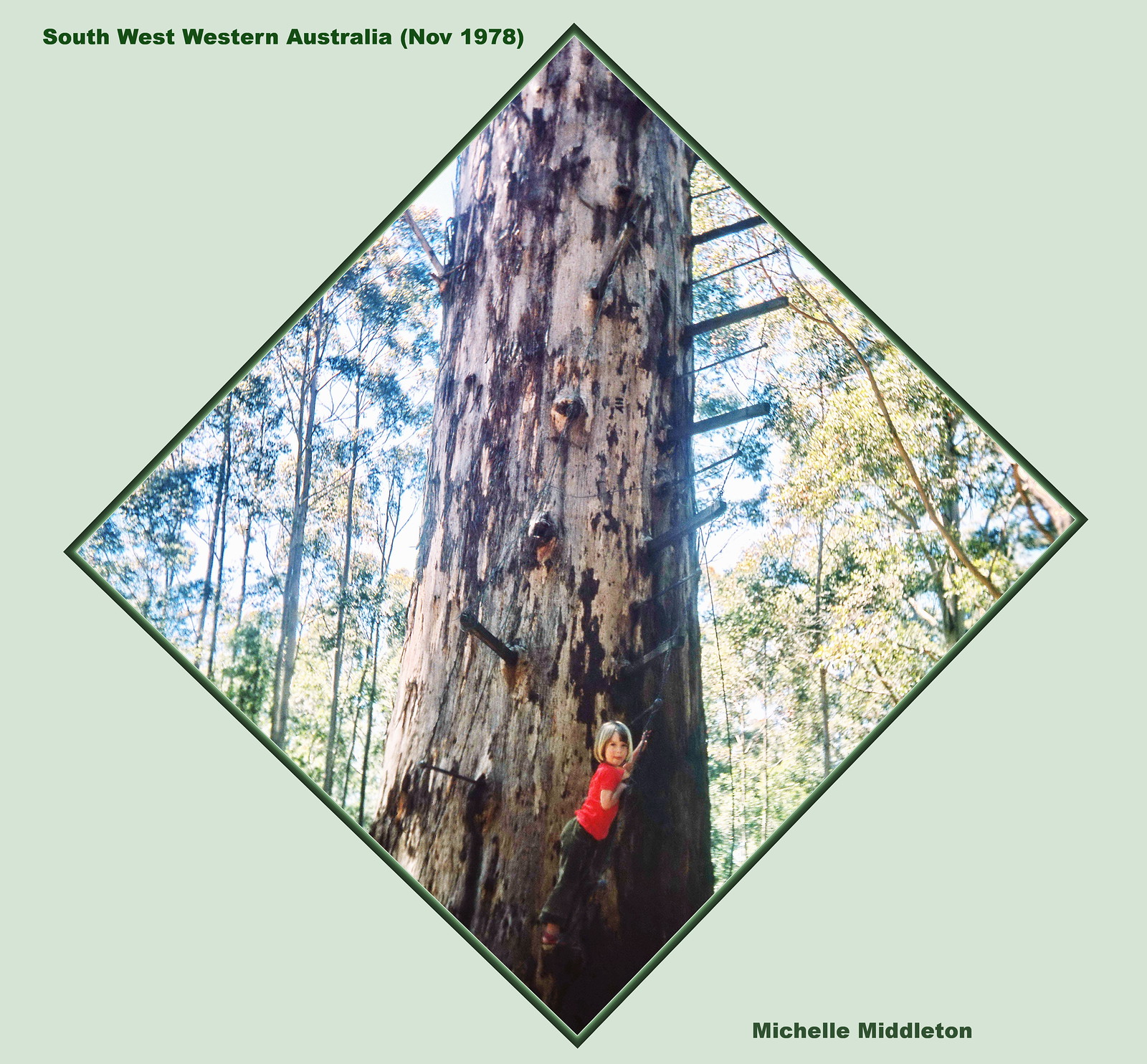A vintage photograph from November 1978, captured in the southwest region of Western Australia, is uniquely framed in a diamond shape. This evocative image portrays a stately, ancient tree, visible partway up, with several broken branches hinting at its age and resilience. The backdrop is filled with a dense forest of soaring, slender trees, which appear leafless and barren, adding to the melancholic tone of the scene. The overall color palette is muted and subdued, with sparse patches of greenery offering subtle hints of life. At the base of the main tree lies a touching focal point—a young girl, approximately four or five years old, gazing into the camera with curious innocence. She is dressed in a vibrant red shirt and blue trousers, her presence injecting a warm, human element into the otherwise stark and timeless forest landscape.